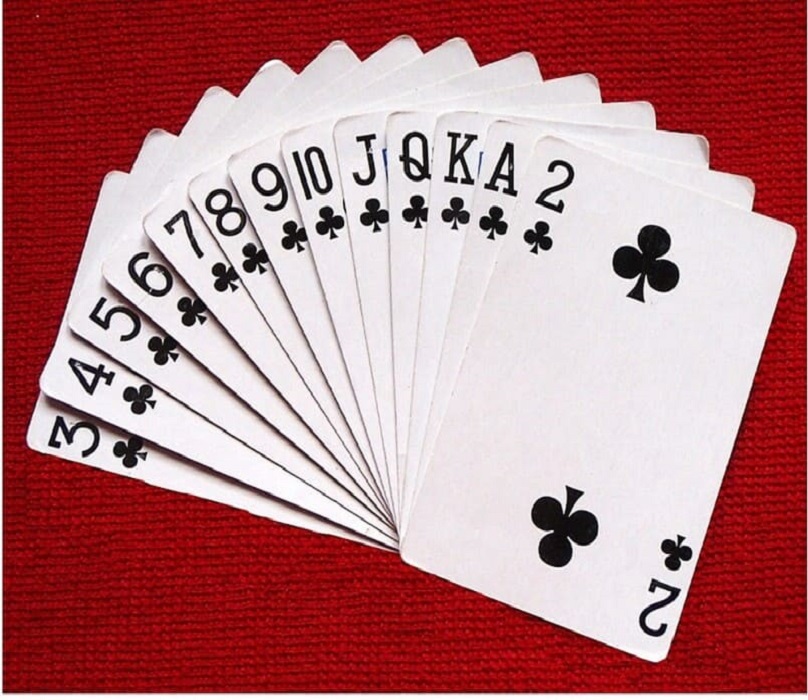A complete set of playing cards from the clubs suit is artistically displayed on a red cloth. The cards are arranged in a fan-like spread, starting with the Two of Clubs followed by the Ace, King, Queen, Jack, Ten, Nine, Eight, Seven, Six, Five, Four, and ending with the Three of Clubs. Each card exhibits a unique degree of wear, evident by the varying bends on the upper right corners, hinting at frequent use. The intricate display captures every card face, emphasizing their unified suit and the character added by their bent edges.